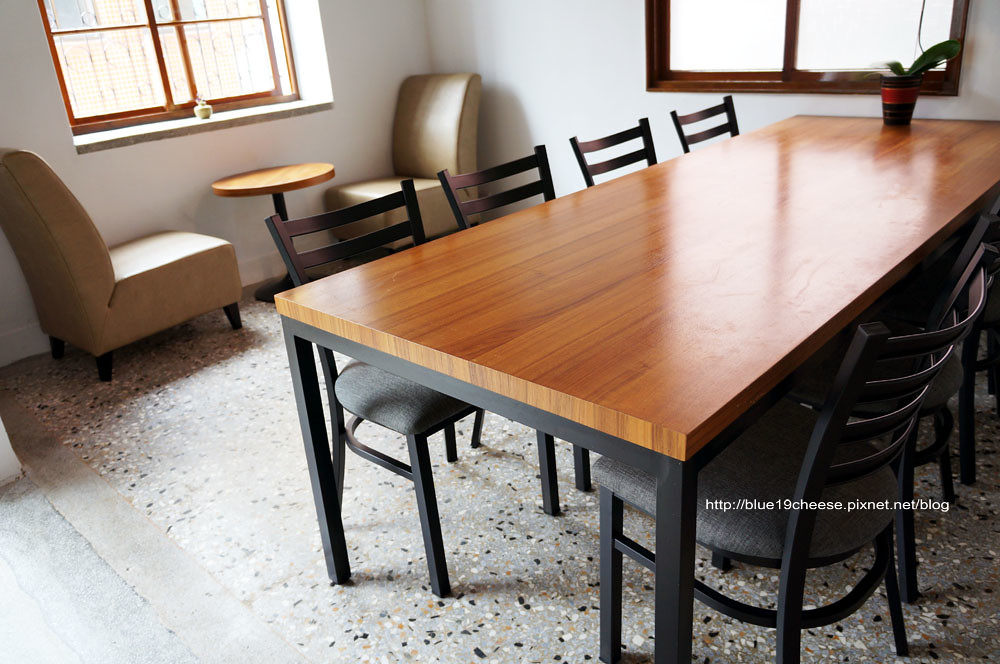This photograph captures the interior of a sunlit cafe with a terrazzo floor featuring a gray marbled appearance with black and white splatters. In the center of the room stands a long wooden table with dark brown streaks, supported by a black metal base. Surrounding this table are eight chairs, each with black legs and backs, and gray cushioned seats. To the left, a smaller, lighter wooden table with a black stand is flanked by two tan lounger chairs. The setting is illuminated by two windows with clear panes and brown wooden frames, offering a view of the sunny exterior. The walls are a plain, light gray, creating a minimalist backdrop. On the floor near the back corner, a URL, "blue19cheese.pixnet.net/blog," is subtly visible, adding a unique detail to the scene.